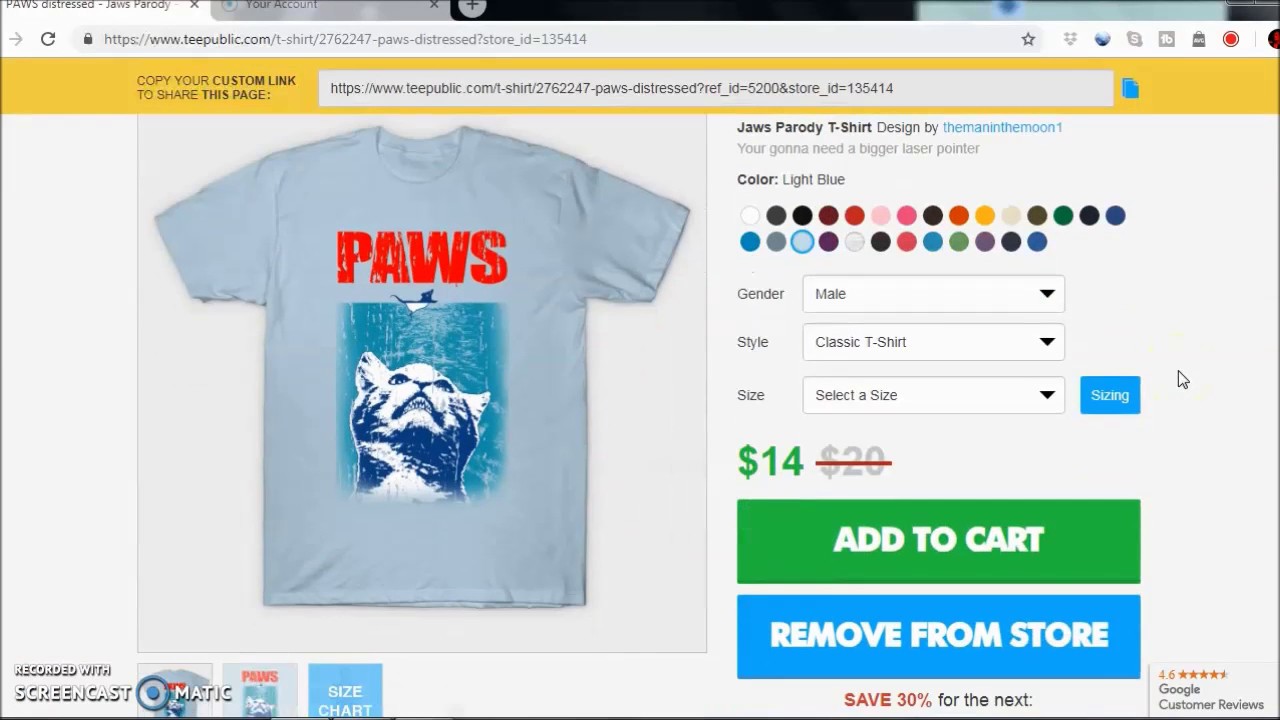This screenshot captures a webpage from a clothing store, showcasing a humorously designed t-shirt. At the top of the page is a yellow search bar. The featured t-shirt is displayed prominently and is light blue, adorned with the word "PAWS" in bold red letters, using the same font as the iconic "Jaws" movie poster. The design depicts a cat emerging from the depths towards a boat at the water's surface, parodying the classic Jaws theme. The shirt is priced at $14, discounted from the original $20, as indicated by the green price listing. The shirt comes in various colors, though the one featured is light blue. It is categorized under "Gender: Male" and described as a "Classic T-Shirt." Shoppers are prompted to select a size from the available options. Below the product details, there is a green "Add to Cart" button, a blue "Remove from Store" button, and a notice offering a 30% discount on future purchases.